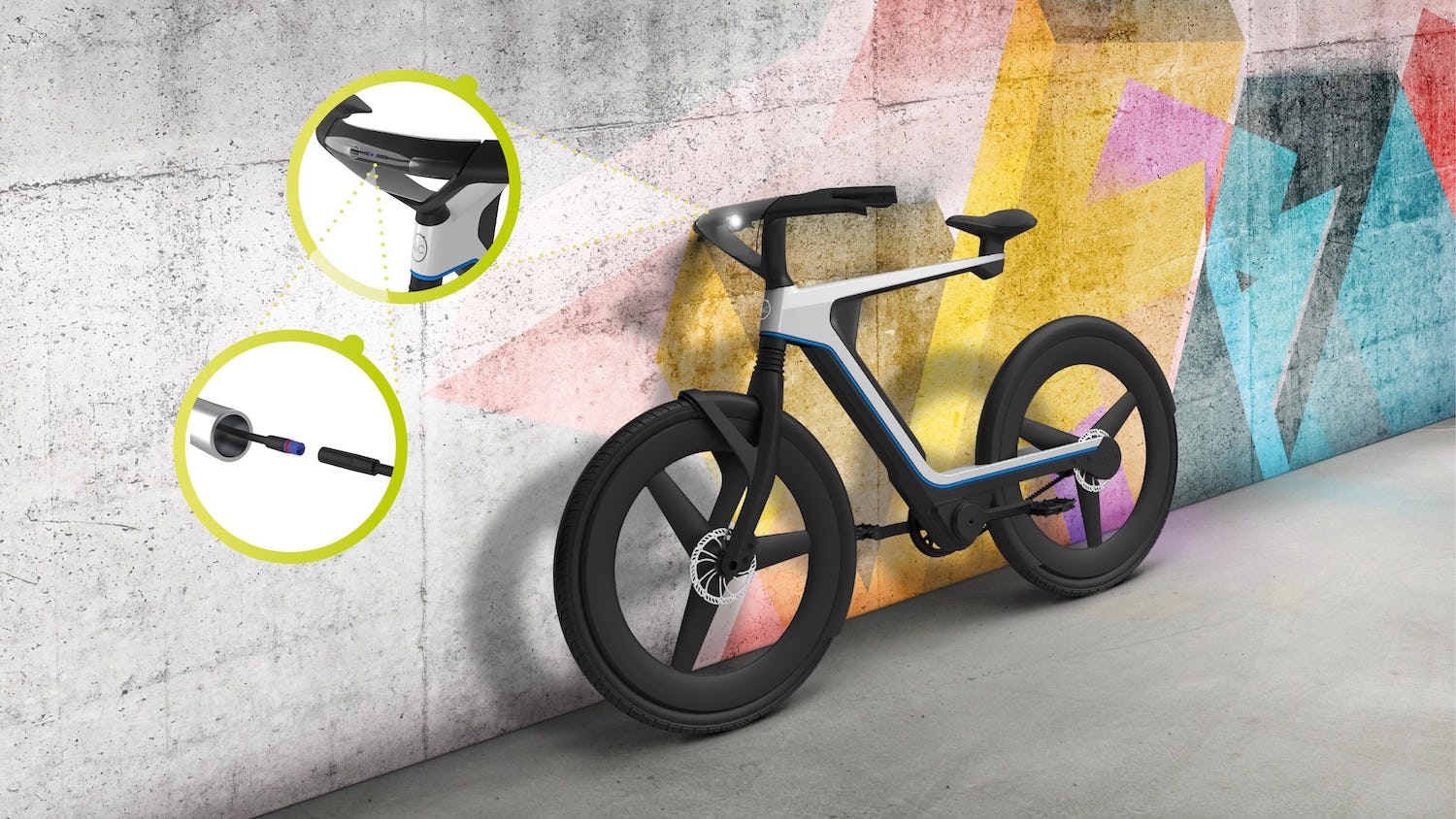This detailed photographic image captures a futuristic two-wheel bicycle leaning against a grey concrete wall adorned with abstract, graffiti-like art. The bicycle features a sleek design with a grey, angular C-shaped frame and a striking open space beneath the seat, which is affixed at the very end of the frame without additional support. The bike's handlebar is a silver U-shape that curves back towards the rider, complementing the black seat. The wheels are solid black with rims supported by three metal spokes, creating a three-pointed star appearance. Detailed inserts within the image show close-up views of the handlebar and the unique braking system, highlighted with green circles and directional arrows. The colorful wall behind the bike includes a purple triangle, golden and black parallelograms, a blue V-shaped element, and various spray-painted shapes in light blue, pink, red, and black, enhancing the modern aesthetic of the scene.